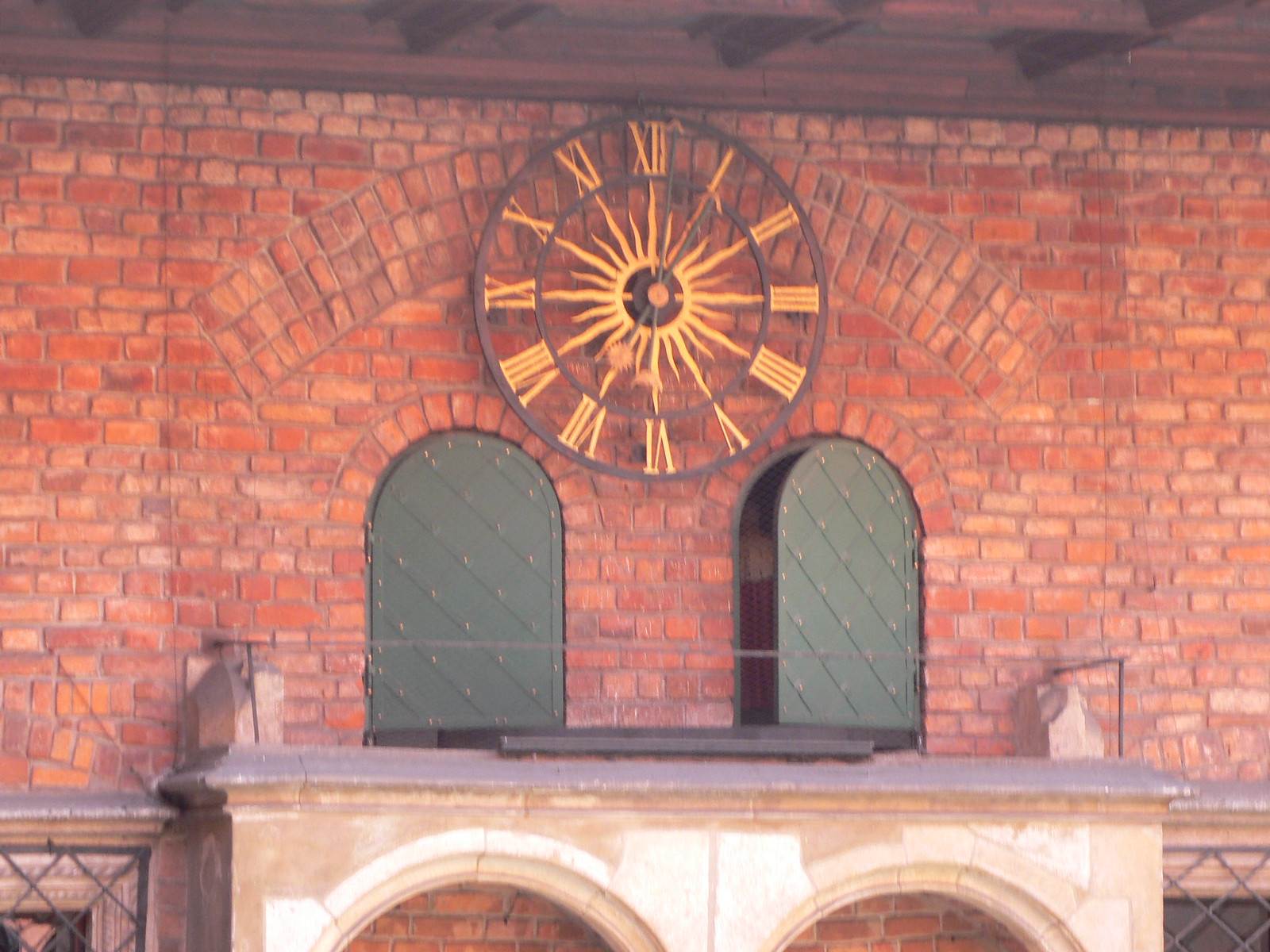This color photograph captures an intricate orange brick wall as its focal point. The horizontal arrangement of bricks is interrupted in the center by an archway pattern, creating a striking visual element. Above this, a dark wooden ceiling adds contrast to the scene. Central to the wall is a decorative clock, embedded within the bricks. The clock features a yellow sunray motif at its center, encircled by a black metal ring. Roman numerals, also in yellow, mark the hours, though the hands, possibly black, are faint and difficult to discern.

Flanking the clock are two green archways resembling doors. The door on the right is slightly ajar, revealing a dark interior. These archways rest upon a gray platform or shelf. Below this, two lighter archways catch the sunlight, adding a touch of warmth to the lower part of the wall. The continuation of the brickwork leads to a metallic fence on the right side, featuring a rectangular trellis design. A similar fence appears on the left. In the bottom left corner, a greyish outline suggests the presence of a window, though details are indistinct. The interplay of architectural elements and varying shades creates a rich and layered composition.